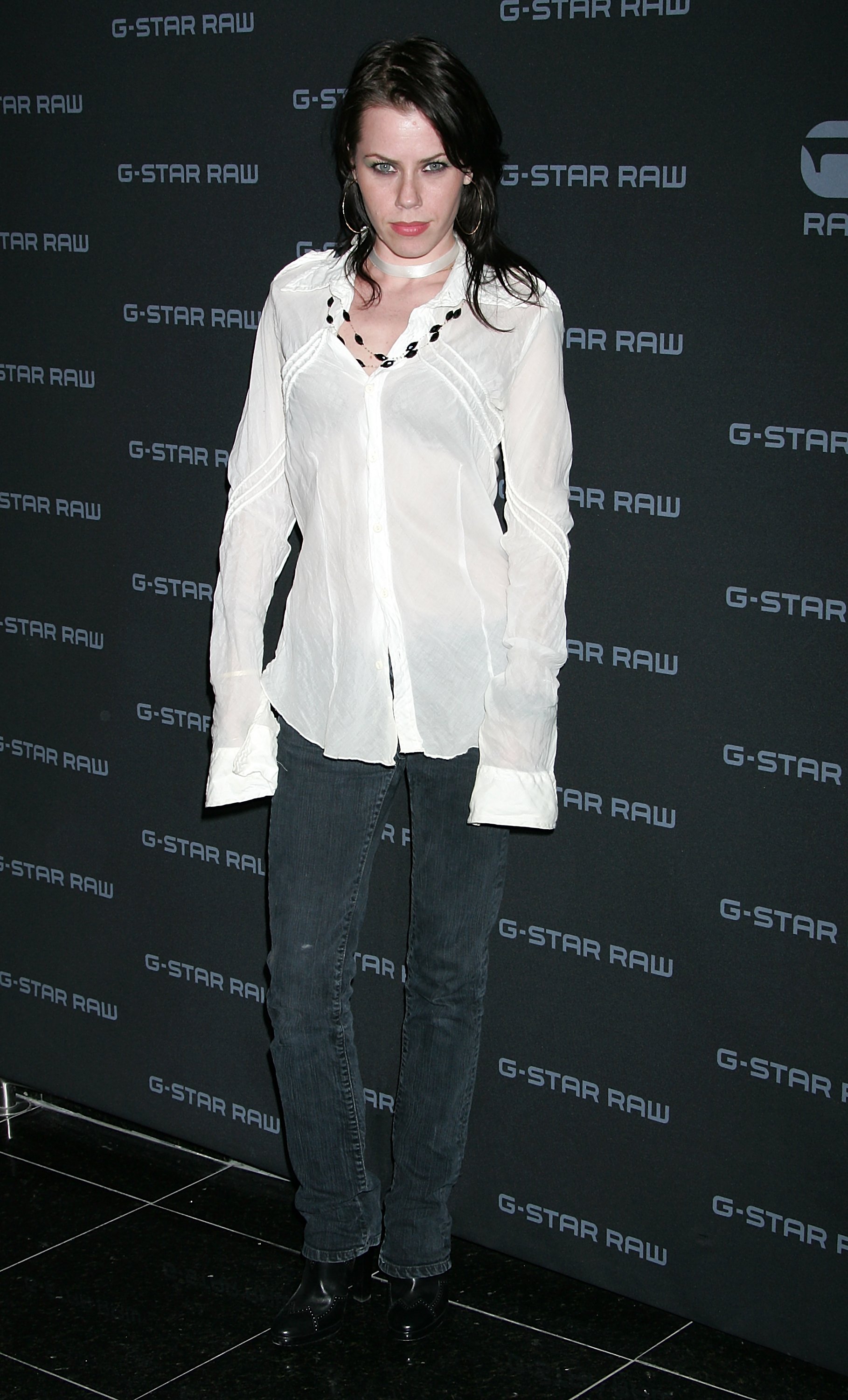In this photograph, an emaciated woman is standing confidently in front of a G-Star Raw banner, which features repetitive white text on a dark background. She is presumed to be a celebrity, possibly Farouk Balk. Her outfit includes a slightly see-through, long-sleeve white blouse that extends beyond her hands, paired with black jeans and black close-toed shoes, potentially boots. She accessorizes with two necklaces; a black one that hangs down to her chest and a silver one around her neck, along with large silver hoop earrings. Her below-the-shoulder length black hair complements her striking red lipstick and defined eyeliner. She stands on a floor made of large black tiles, staring directly into the camera.